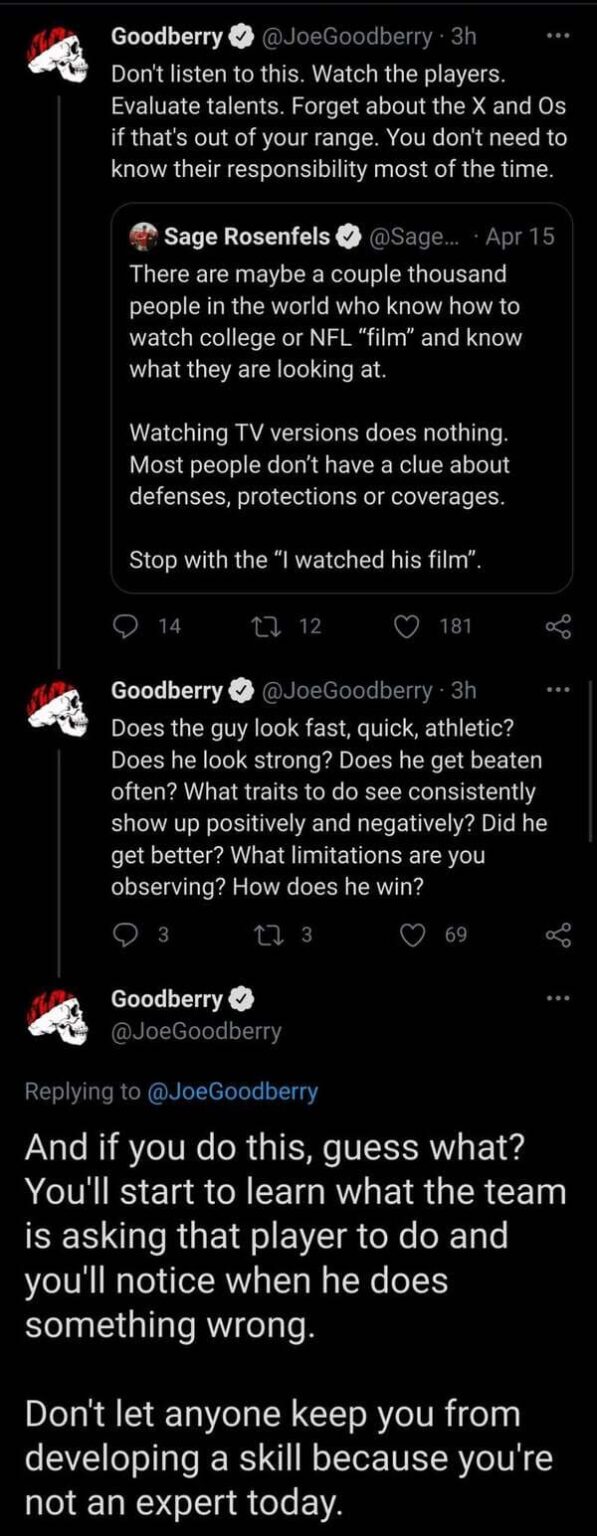The image falls under the category of "Websites" and features a dark-themed background with a sleek, user-profile interface. Situated at the top is a small profile picture depicting a skull adorned with a red and black cap. Next to this image, it reads "Goodberry" with a verified icon, followed by "@Joe Goodberry."

Below this, there is a succinct yet focused message advising viewers to prioritize evaluating players' talents over understanding complex strategies (X's and O's), stating that lacking detailed knowledge about the players' responsibilities is acceptable for most fans.

The message transitions into a tweet from Sage Rosenfels, identified by the handle "@Sage," who adds to the conversation. Rosenfels emphasizes that only a select few individuals can properly analyze college or NFL film beyond mere TV broadcasts. He points out that many lack an understanding of defenses, protections, or coverages, and advises against forming opinions based solely on watching film superficially.

Joe Goodberry’s response suggests a more straightforward approach to evaluating players by observing physical traits such as speed, agility, athleticism, and strength. He advises looking for consistency in positive and negative traits, assessing if the player shows improvement, identifying limitations, and understanding how they succeed on the field. By repeatedly doing this, one can gradually learn what the team expects from the player and more accurately identify mistakes.

The underlying message encourages self-improvement in football evaluation skills without feeling intimidated by initial lack of expertise.